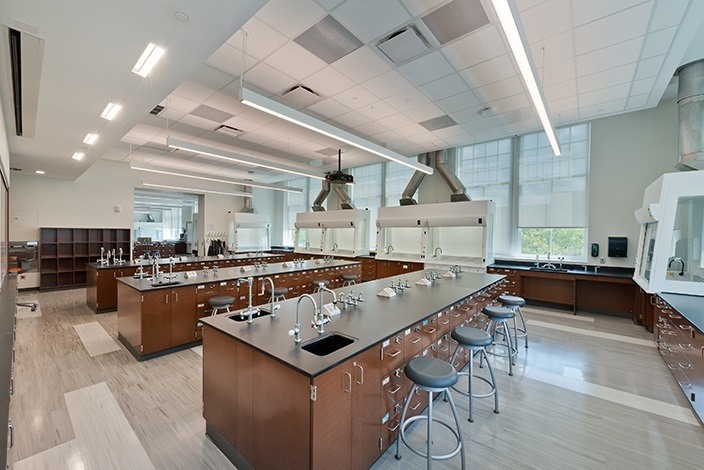This indoor photo prominently features a classroom or laboratory setting with a clean, organized layout. Dominating the room are long tables with shiny gray surfaces, complemented by brown cabinets, each adorned with sleek silver metal handles. These cabinets, which line the sides of the room, also feature small rectangular sinks topped with faucets, and there appear to be three such sink setups visible. The floor is a light wood-tone, almost off-white, enhancing the room's brightness. Tall windows line one of the white walls, allowing ample natural light to stream in. Suspended from the white ceiling are multiple long light fixtures and additional ceiling lights. The ceiling also has noticeable air vents. Black stools are strategically placed either on the tables or next to the cabinets. A seemingly empty bookcase or bookshelf is also part of the room's furnishings, adding to the overall sense of spaciousness and utility in this well-equipped educational or laboratory environment.